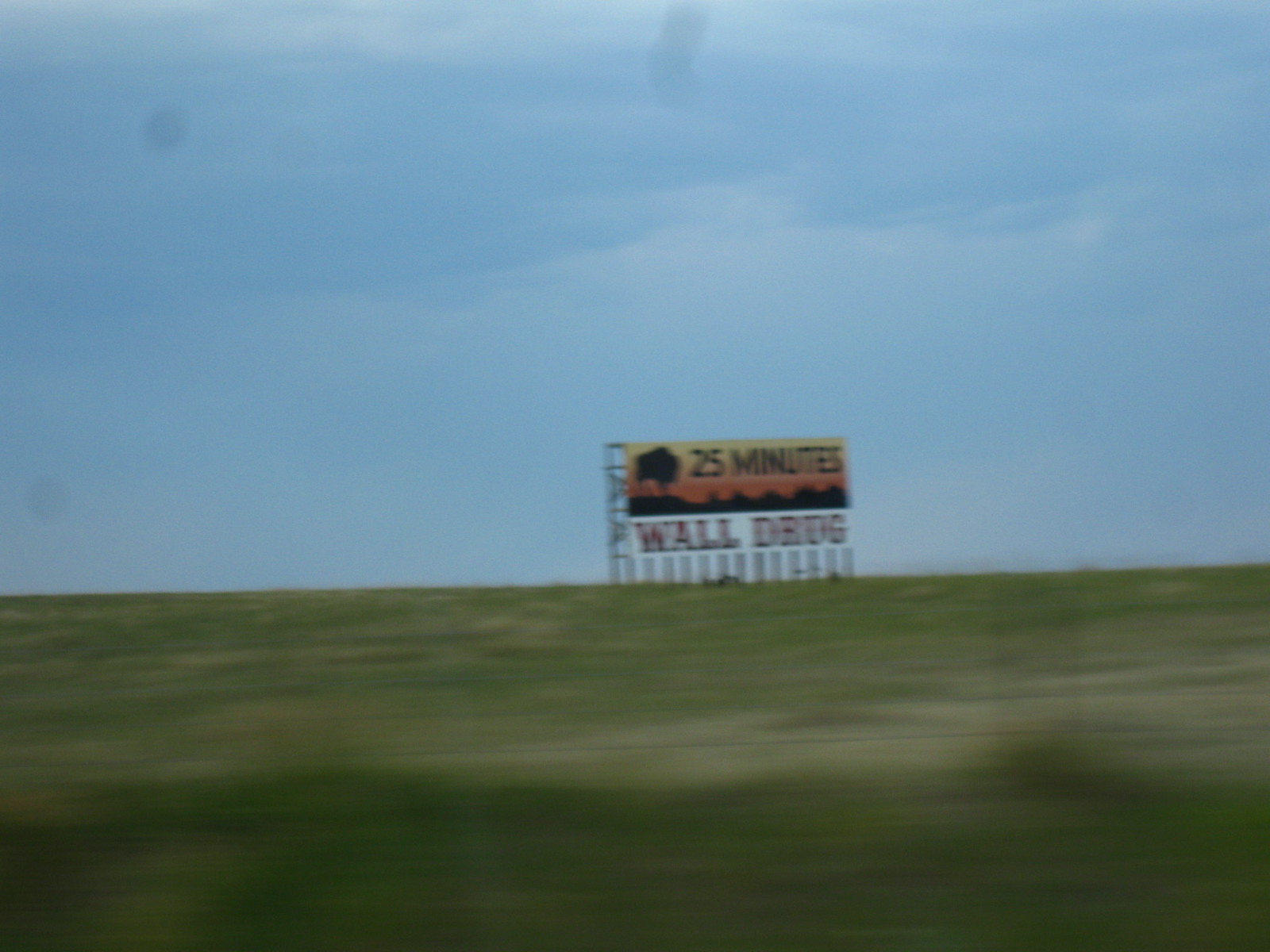This slightly blurry and out-of-focus color photograph, seemingly taken from a moving car, captures a large rectangular billboard set in an expansive, flat grassy field. The green expanse is slightly blurred, giving a sense of motion. Towering above the landscape is a clear yet slightly hazy blue sky. The billboard itself is divided into two distinct sections. The upper part features a golden-red-yellow background with a black silhouette of a bison on the left and the words "25 minutes" boldly inscribed in black. Below, on a white background, the billboard prominently displays "Wall Drug" in red letters. Supporting the billboard are several visible structures. The scene is devoid of other structures or trees, isolated against the vast, open landscape.